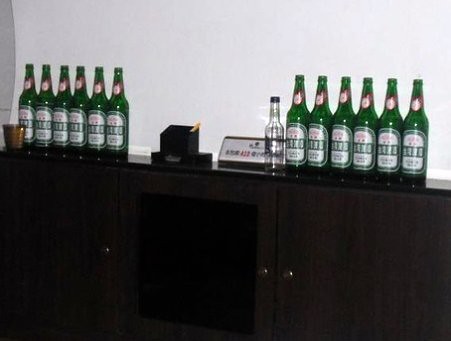This image portrays a dark wood floor cabinet positioned against a light blue wall, where the top half of the wall is visible. The cabinet features three distinctive doors: the left door is solid brown with a silver handle on the right, the middle door is black with a dark brown border and a handle on the right, and the right door is solid brown with a handle on the left, topped with a thin black border. Atop this cabinet is a neatly arranged collection of green beer bottles, each adorned with a label featuring green borders and unreadable white lettering. There are six bottles aligned on either side of the cabinet, separated by a small black box containing what appears to be a cigarette or a pencil, and a desk nameplate. Additionally, a silver shot glass is placed on the left, and a glass bottle, possibly for liquor, is situated in front of the nameplate, creating a symmetrical display of the bottles and items on the shelf.